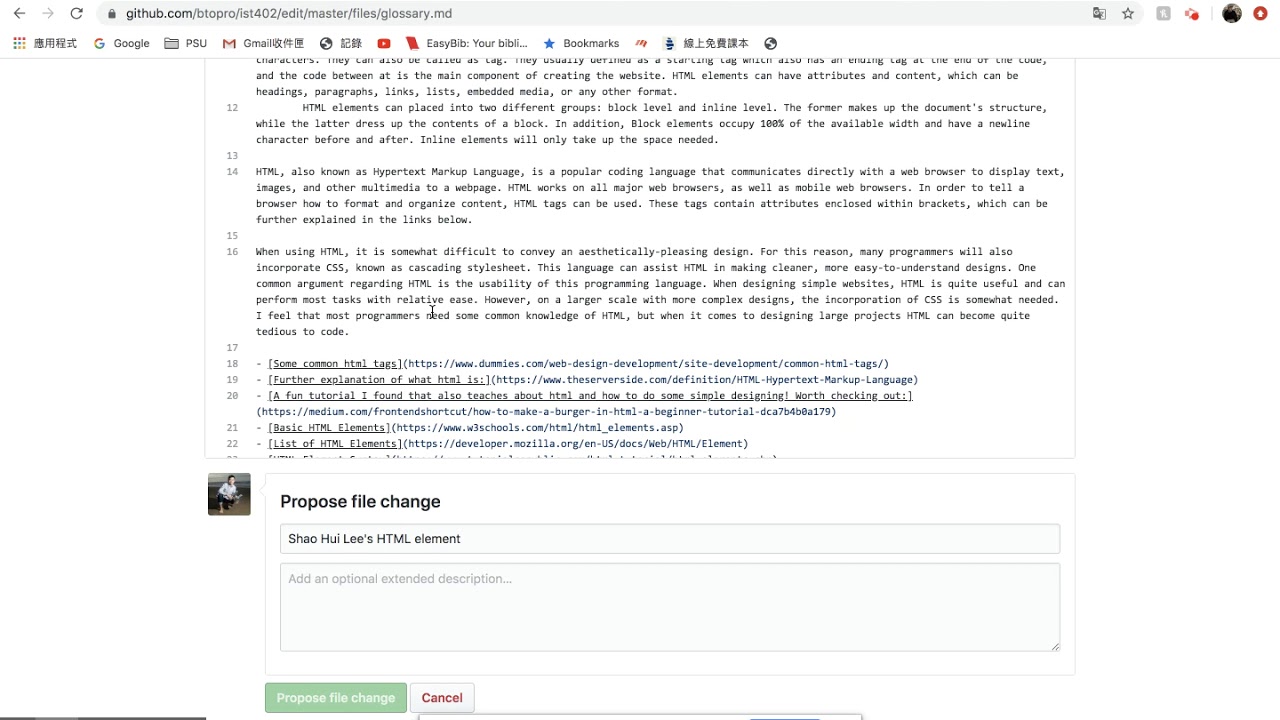A detailed webpage caption for a GitHub repository screenshot:

The screenshot captures a web page interface from GitHub, specifically located at "github.com/btopro/ist402/edit/master/files/glossary.md". At the top of the page, the standard navigation icons are visible, including the left and right arrows and a refresh symbol. These elements indicate it's a typical web browser view. To the right of the URL, familiar symbols for various browser functions are displayed.

Immediately below, a horizontal toolbar features the Google emblem—represented as a 3x3 grid of multi-colored dots. Adjacent to this are Asian characters followed by the word "Google". Next, there is an icon of a folder labeled "PSU", followed by the Gmail symbol labeled "Gmail" with accompanying Asian text. It continues with another icon that appears to signify an internet browser, also labeled in Asian script. Additional icons in this toolbar include the YouTube logo, a link for "Easy Bib", and a bookmarks icon marked by a blue star.

Further down, the main content area of the page shows information pertaining to the file being edited. This section includes a styled box with rounded corners displaying a user's avatar. Next to the avatar, another box indicates that the user is proposing a change to the file. Text within this box reads "Proposed file change" and provides the user's name, followed by an "HTML element" label. Below this, a prompt invites the user to "Add an optional extended description". 

At the bottom of this section, two interactive elements are presented: a green button labeled "Propose file change" in white text and, beside it, a white button with red text that reads "Cancel".